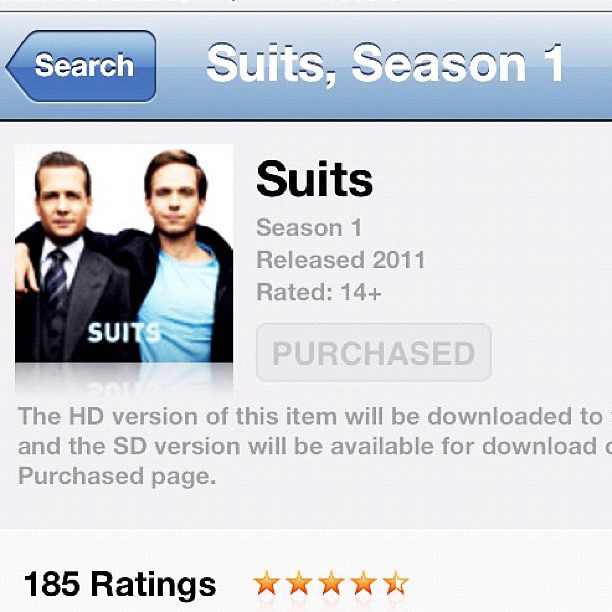This is an advertisement for the TV show "Suits," specifically highlighting Season 1. At the top of the screen, there is a blue bar with a search arrow on the left. To the right, it displays "Suits, Season 1" in white font. Beneath this, an image features two men sitting closely, with one man having his arm around the other's shoulder, reflecting the camaraderie of the show's main characters.

To the right of the image, the text "Suits, Season 1, released 2011, rated 14+" is displayed, indicating the show's release year and age rating. Below this, there is a rectangular bar that says "Purchase," suggesting that the user has already bought the series. A partial text visible reads, "The HD version of this item will be downloaded to..." and "...the SD version will be available for download," but the rest of the information is cut off.

The page also indicates that there are 185 ratings for this season, with an impressive average rating of 4.5 stars. The lettering on the page is presented in light gray on a lighter gray background, maintaining a sleek and modern aesthetic.